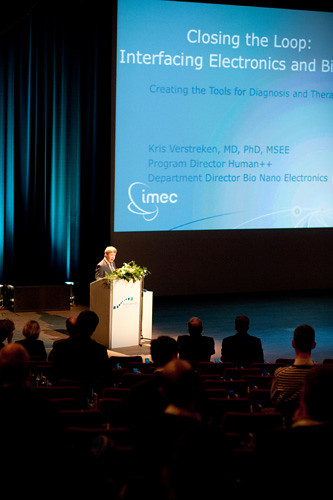The photograph, a vertically aligned rectangular image, captures a scene from an event, likely a medical conference. Taken from the back of the audience, the image prominently features a man in a gray suit with short, light-colored hair, standing just to the left of center on a large stage. He is illuminated by a spotlight as he stands at a white and brown podium adorned with a selection of green leaves at the top. The face of the podium is decorated with blue dots across the center. Behind the man, a dark blue curtain forms the backdrop.

To the upper right of the image, a projection screen displays text on a blue background. The white text reads, "Closing the Loop, Interfacing Electronics," followed by partially obscured writing. Beneath it, in blue text, the screen says, "Creating the Tools for Diagnosis," with the remainder also partially cut off. The lower part of the screen identifies, in blue text, "Christopher Staken, MD, PhD, MSEE," along with his titles as "Program Director, Human++, Department Director, Bio Nano Electronics." The bottom left-hand corner of the projection screen features a white logo that reads "IMEC." The foreground of the image shows the backs of several audience members' heads, indicating that the photo was taken from an auditorium's seating area.